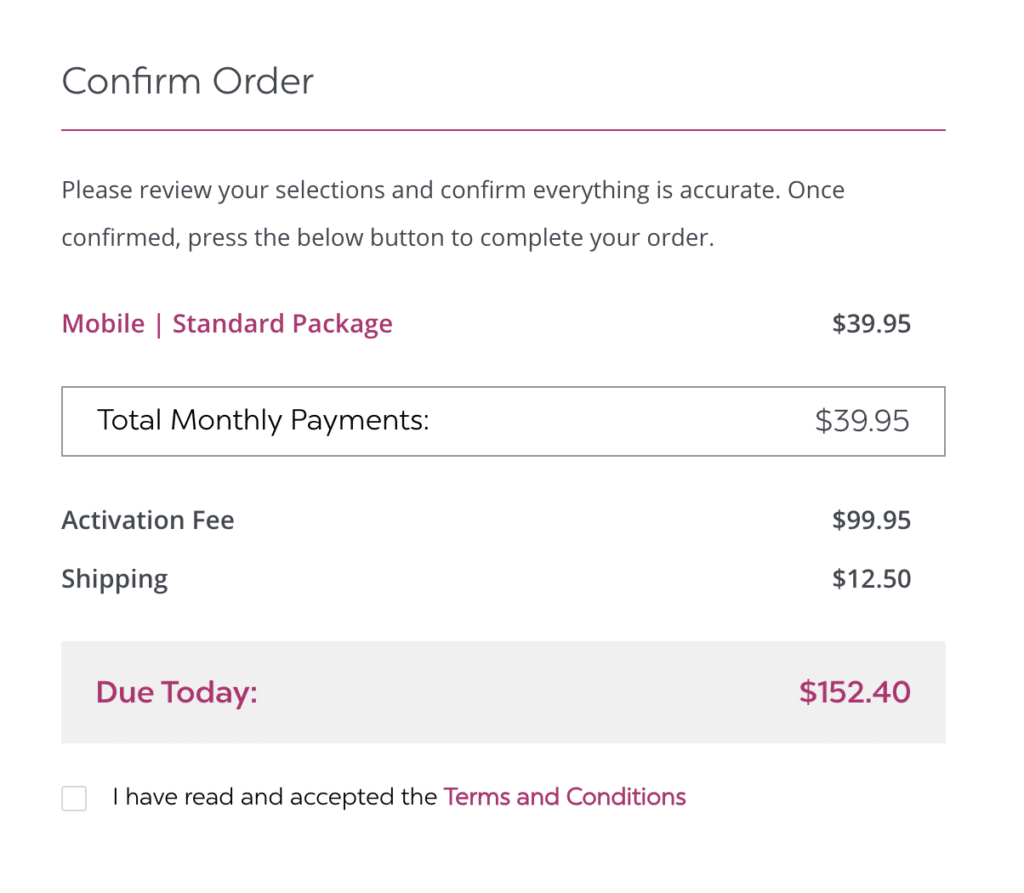The image features a confirmation screen set against a white background, with text in a mix of black, gray, and pinkish fonts. 

At the top, prominently displayed in black or pinkish-colored text, are the words "Confirm Order." Directly beneath this title is a thin pinkish line, followed by an instructional note in gray text, which reads: "Please review your selections and confirm everything is accurate. Once confirmed, press the button below to complete your order."

Below this note, a detailed breakdown of the order's contents and charges is provided:
- "Mobile Line Standard Package" is highlighted in pink, followed by the price "$39.95" in black.
- "Total Monthly Payment: $39.95" is also in black, enclosed within a bordered box.
- Additional charges are listed as follows: "Activation Fee: $99.95," and "Shipping: $12.50."
- The total amount due today, "$152.40," is emphasized in pink.

Near the bottom of the screen, there is an unchecked box next to the statement: "I have read and accepted the terms and conditions," with "terms and conditions" displayed in pinkish text.

The overall color scheme of the screen includes tones of black, gray, pinkish, and white, but there are no additional contextual elements indicating whether this is displayed on a phone, website, or application.